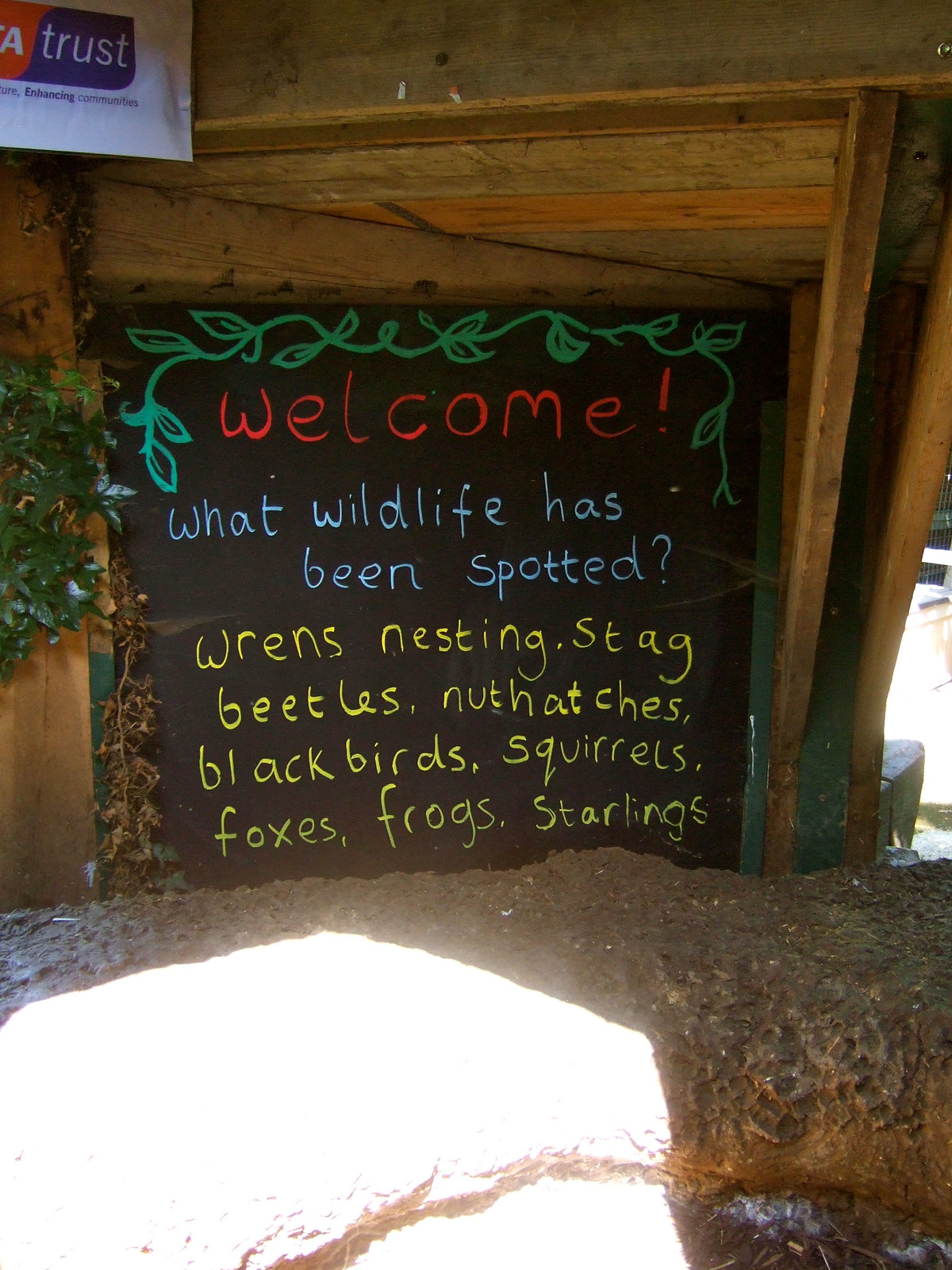The image depicts an outdoor area featuring a wooden shelter with a black chalkboard framed by wooden walls and support beams. The blackboard, adorned with painted vines and leaves at the top, is handwritten with various colored markers. The red text at the top reads "Welcome," followed by light blue text asking, "What wildlife has been spotted?" Underneath, in yellow text, it lists wildlife sightings: "Wrens nesting, Stag beetles, Nuthatches, Blackbirds, Squirrels, Foxes, Frogs, Starlings." The surrounding area includes a small concrete barricade and vegetation on the left side, with leaves from a bush or low tree peeking into the frame. The setting appears shaded overall, except for a small, brightly lit section in the bottom left corner, suggesting the presence of sunlight filtering through. The scene evokes a natural, perhaps park-like or zoo environment.